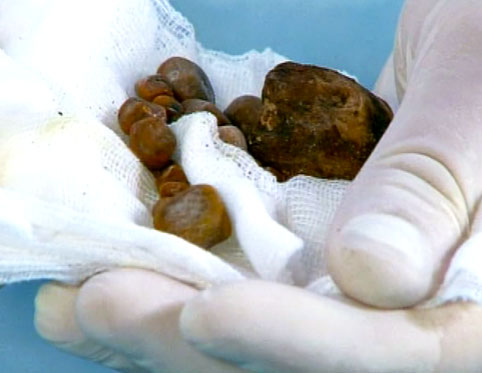The image depicts a close-up of a left hand, belonging to a white person with trimmed nails, cradling a piece of very bright white gauze against a blue background. The gauze is slightly crumpled in the palm, with several roundish, brownish objects placed on it. These objects, varying in size but mostly small and possibly greenish-brown, appear to be under examination. The perspective and setting, combined with the use of gauze, suggest a medical context—potentially items removed surgically, such as stones or tumors. Despite the lack of clear gloves on the hand, the scenario hints at a meticulous, closely observed procedure.